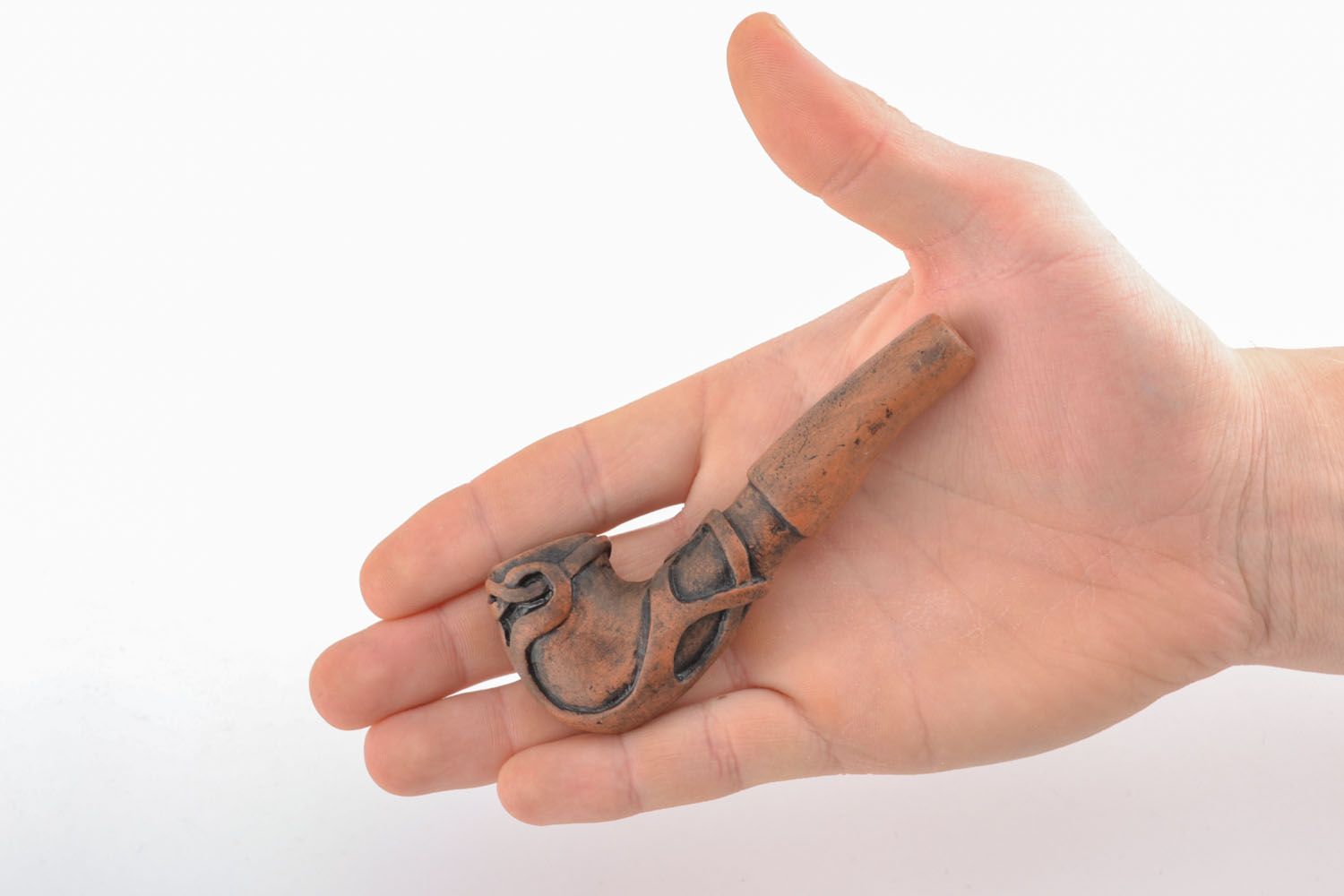This color photograph captures the right hand of a fair-skinned individual, likely a man, extending from the right side of the image against a plain white backdrop. The hand is palm-up, cradling a small smoking pipe, which appears to be carved from either brown wood or terracotta-like clay. The pipe is short, with the bowl situated towards the left side of the hand and the mouthpiece towards the right. The bowl features an intricate, vine-like Celtic design etched around it, accentuated with black edging, while the mouthpiece remains flat and solid. The upper part of the stem is notably thick, adding to the pipe's earthy and robust appearance.